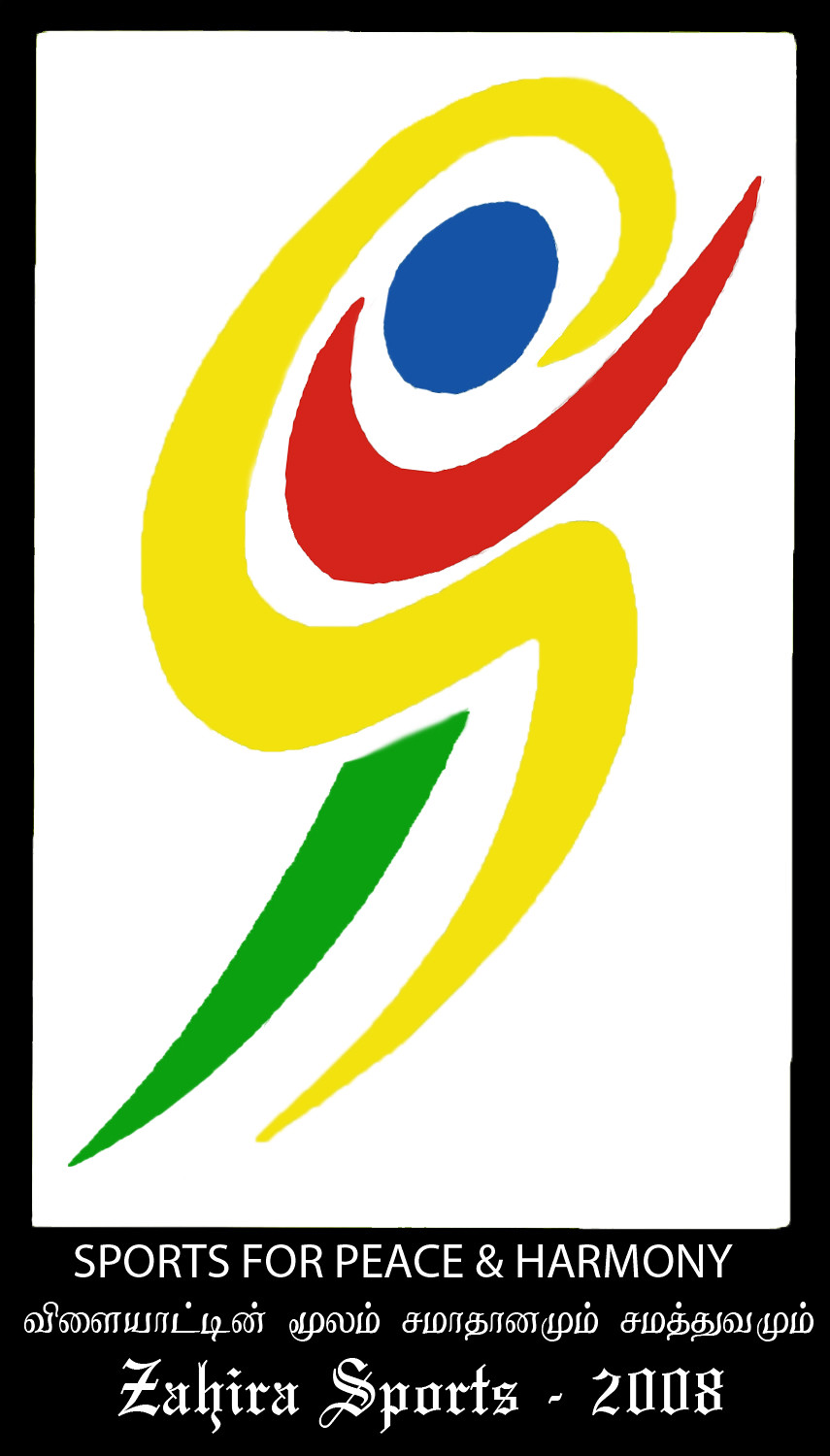This photograph features an advertisement with a logo framed in black against a white background. The logo intricately combines various colored shapes to create a stylized representation of a person running. The head is depicted as a blue circular dot at the top, while a red circular check mark forms the arm. A yellow line curves in an S-shape from top to bottom, representing the body, and a green line, shaped like an upside-down blade of grass, symbolizes the legs. Below this vibrant design, the text "Sports for Peace and Harmony" is displayed in white letters within the black frame. Additionally, there is an inscription in an unspecified foreign language, followed by "Zahira Sports, 2008." This artwork appears to be part of a promotional piece highlighting a special sporting event focused on fostering peace and harmony through sports.